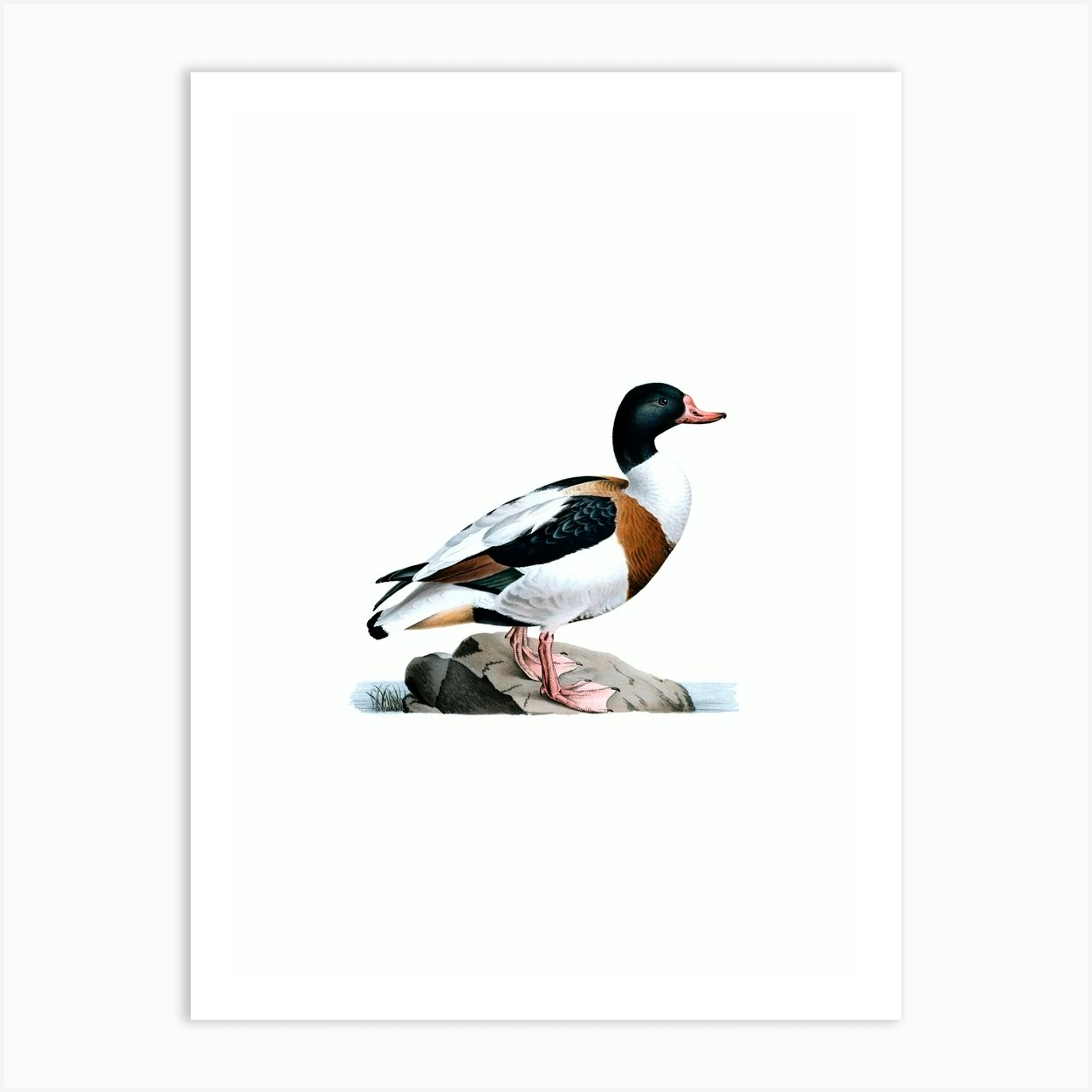This image depicts a meticulously detailed print that resembles a painting of a multicolored duck, possibly a mallard, standing on a rock. The duck, facing right, is set against a completely white background, creating a sharp contrast that emphasizes its form and colors. The duck’s head is a deep hunter green, transitioning to a white neck and upper chest. Its breast is tan, and its underbelly is white. The wings match the head with the same hunter green hue, tapering off into brown tips. The duck’s webbed feet are flesh-toned, firmly planted on the rock, giving the impression it is peering attentively into the water below. The surrounding environment includes subtle details of water and a hint of grass beneath the rock. The print itself occupies only about a third of the white poster board it’s on, leaving a very large border and providing a formal, elegant appearance without any additional framing. The duck's pose and expression convey a sense of focused contemplation, enhancing the overall serene and poised mood of the artwork.